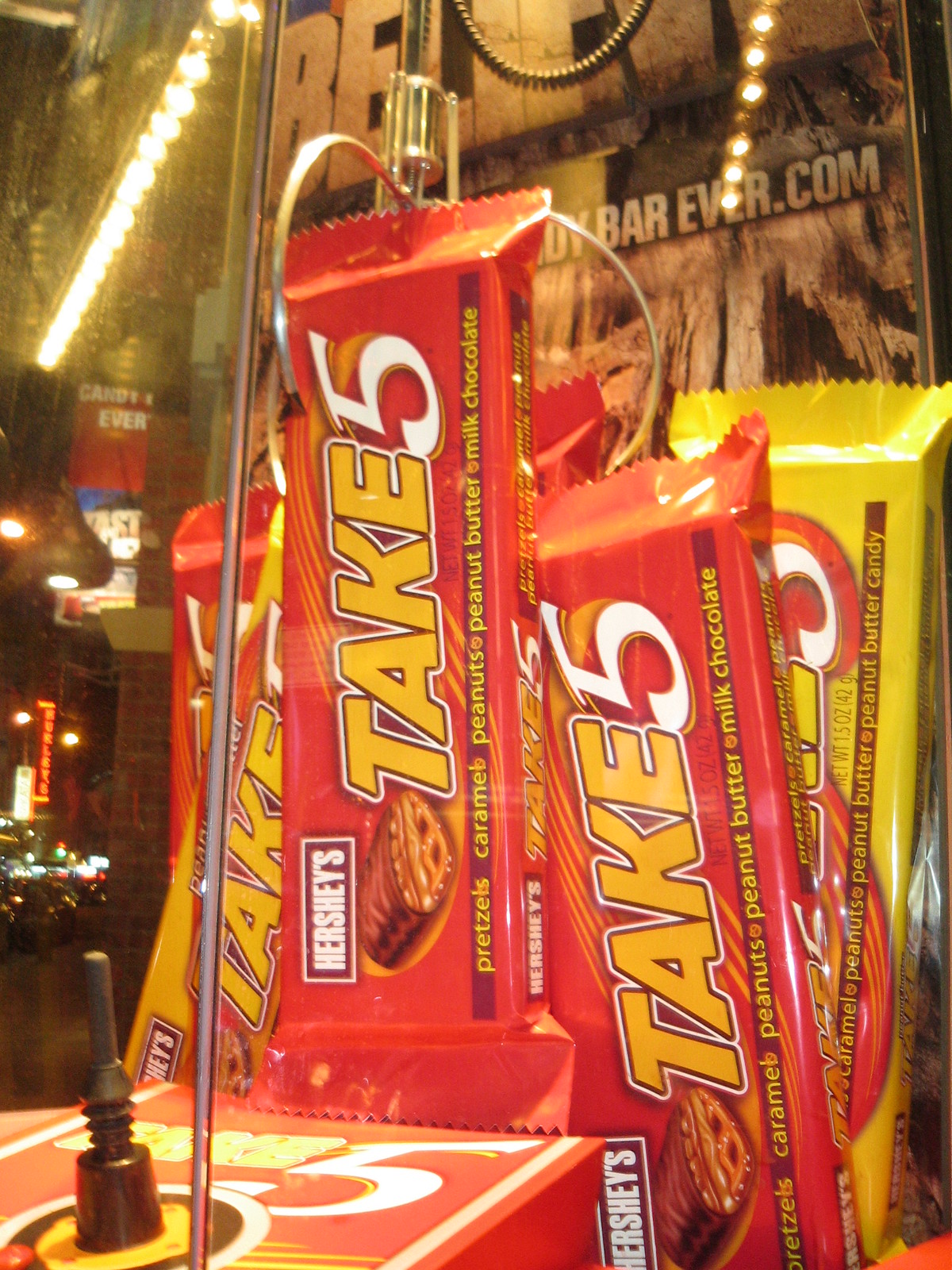The color photograph captures a display of Hershey's Take 5 chocolate bars, viewed through a glass resembling that of a museum exhibit or a claw machine arcade game. The candy bars are neatly arranged upright within the case. Majorly encased in a vibrant orange packaging, the Take 5 bars prominently display the Hershey's logo vertically in white on a brown background along the left side. Beneath the large yellow "Take" text coupled with a white number "5" detailed with a dark red and outer white-red border, there is a strip listing the delectable ingredients: "pretzels, caramel, peanuts, peanut butter, and milk chocolate" in yellow text on a dark red background. An illustrative cross-section of the bar shows off the layered fillings. Additionally, a thin banner featuring "BarEver.com" and "Candy Ever" runs beneath the chocolate bars, and a small lever or bell peeks out from the bottom left of the frame. The overall intricate arrangement inside the glass silently invites closer inspection of this indulgent treat.